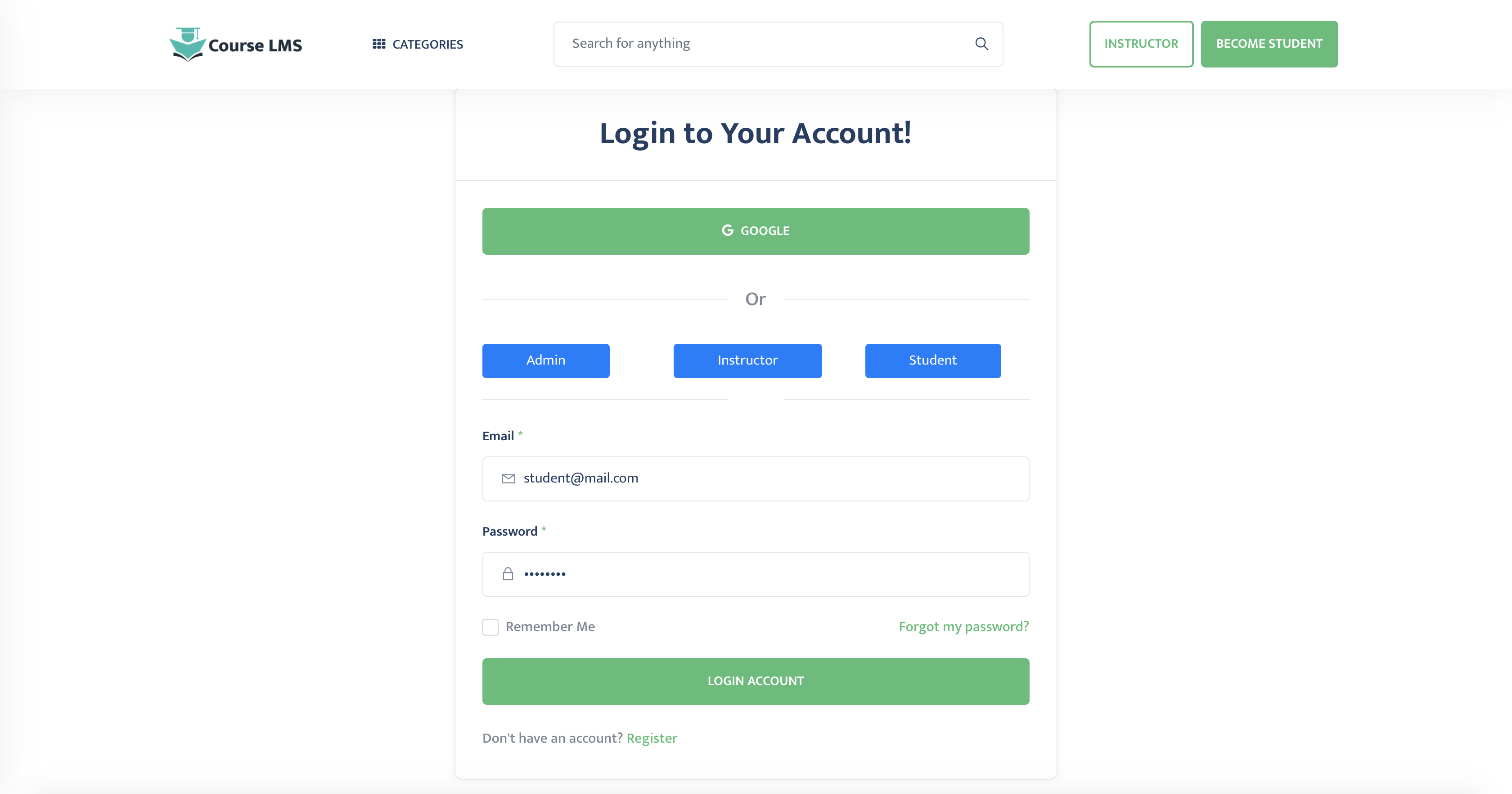On a white background, the layout prominently features "course LMS" with "LMS" capitalized. At the top, there is a hamburger icon for the menu and a search bar with a magnifying glass icon. Below, there's a white rectangle with "Instructor" written inside, and a green rectangle with "Instructors" written in white.

Additionally, there is a white rectangle with "Become Student" in green and another green rectangle containing "Login to your account" in blue text. This section includes options for logging in with Google, separated by "OR," followed by admin, instructor, and student login options, each in their respective blue rectangles with white text.

The form fields include a box for entering your email address labeled "Email," a box for the password with placeholder dots, and a "Remember me" checkbox. There's also a "Forgot my password?" link in green with a question mark. At the bottom, there is a green rectangle with "Login Account" written in white text. For new users, "Don't have an account?" is written above a green "Register" link.